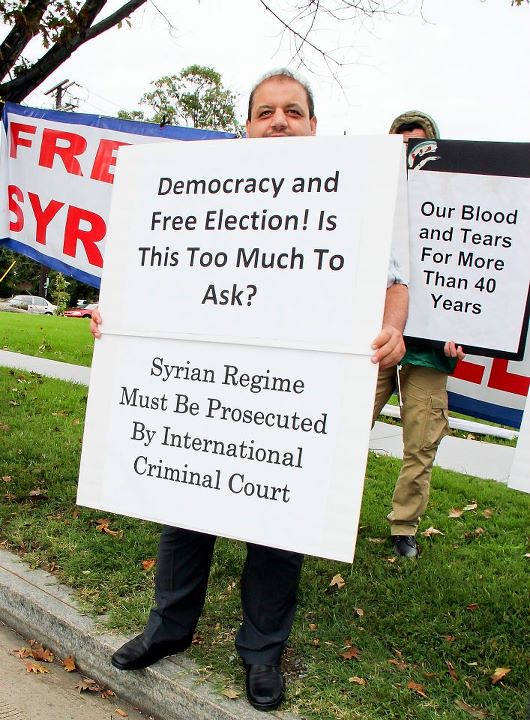In a hazy, overcast day, a photograph captures a vivid scene of a protest or demonstration set against a backdrop of grass with scattered leaves, bare trees, and utility poles. At the center of the image, a man stands on a narrow strip of grass beside a curb, holding a large white sign that obscures much of his body, revealing only his face from the nose up and his lower legs dressed in black pants and shoes. His sign, covered in gray print, proclaims: "Democracy and Free Election. Is this too much to ask? Syrian regime must be prosecuted by International Criminal Court." 

Just behind him, a second man, partially concealed, holds a sign that reads: "Our blood and tears for more than 40 years." He is clad in khaki pants and a hoodie. The sky above is a solid white, adding to the hazy atmosphere. In the background, other protesters hold signs, including a partially visible large banner with the letters "F-R-E-S-Y-R" in red text on a white background with a blue border. Cars can be seen parked at a distance, reinforcing the sense of public outcry captured in the image.